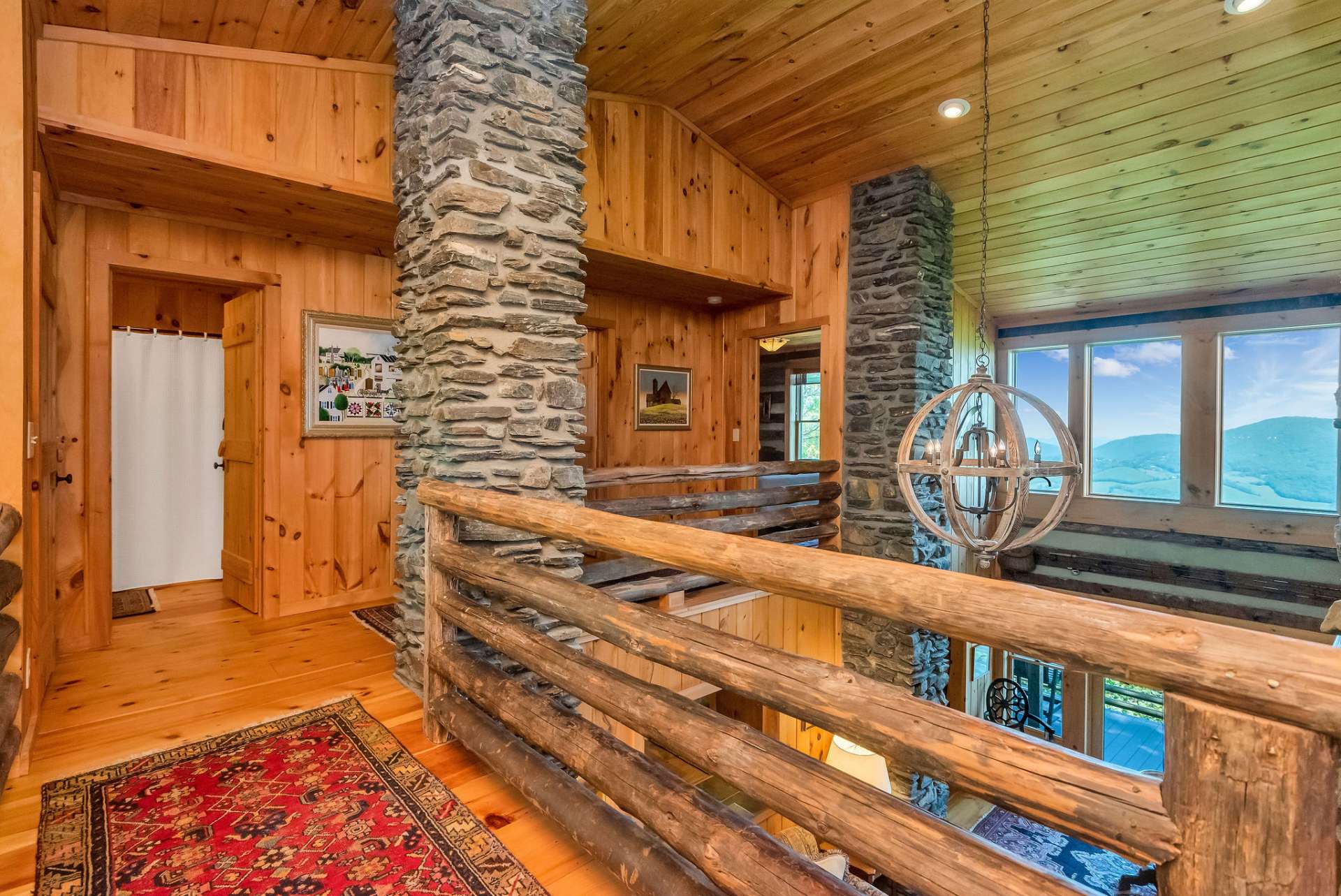A photograph capturing the second floor of a luxurious log cabin, showcasing an elegant blend of wood and stone elements. The space boasts wood flooring, walls, and a cathedral ceiling adorned with recessed circular lights. Two imposing stone pillars stretch from floor to ceiling, anchoring the room. A red Persian hallway rug runs along a wooden walkway on the left, leading to an open wooden door where a white shower curtain is visible. The hallway walls are decorated with framed photographs. On the right-hand side, large windows offer views of a scenic landscape, possibly a lake or mountains, enhancing the cabin's natural charm. A spherical chandelier hangs prominently at eye level, illuminating the open-concept design that overlooks the first floor, separated by horizontal log railings fixed between the stone columns.